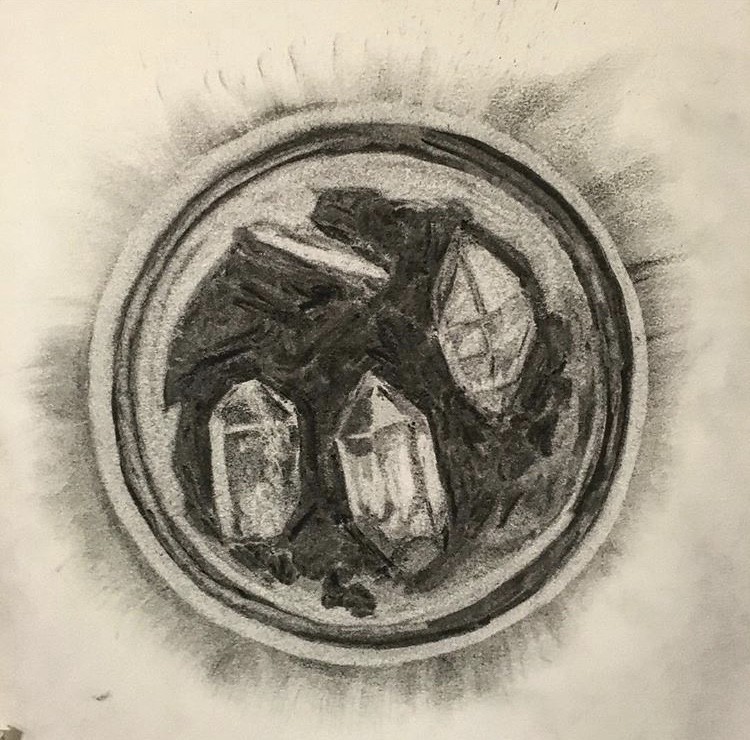The drawing depicts a detailed inside view of a cup filled with soda, masterfully hand-drawn using pencil or charcoal on slightly off-white paper. The liquid inside the cup is shaded in a deep black, contrasting starkly with the clear ice cubes floating within, creating a striking visual effect. In the middle of the cup, several gemstones or diamond-shaped pieces are intricately drawn, featuring careful shading to highlight their indentations and dimensions, with one prominent diamond lying on its side. The outer rim of the cup is defined by multiple circles with varying degrees of shading from black to light gray, and the entire composition is surrounded by radiating black and gray lines. The bottom left corner of the paper also has notable dark smudges, adding to the depth of the piece.